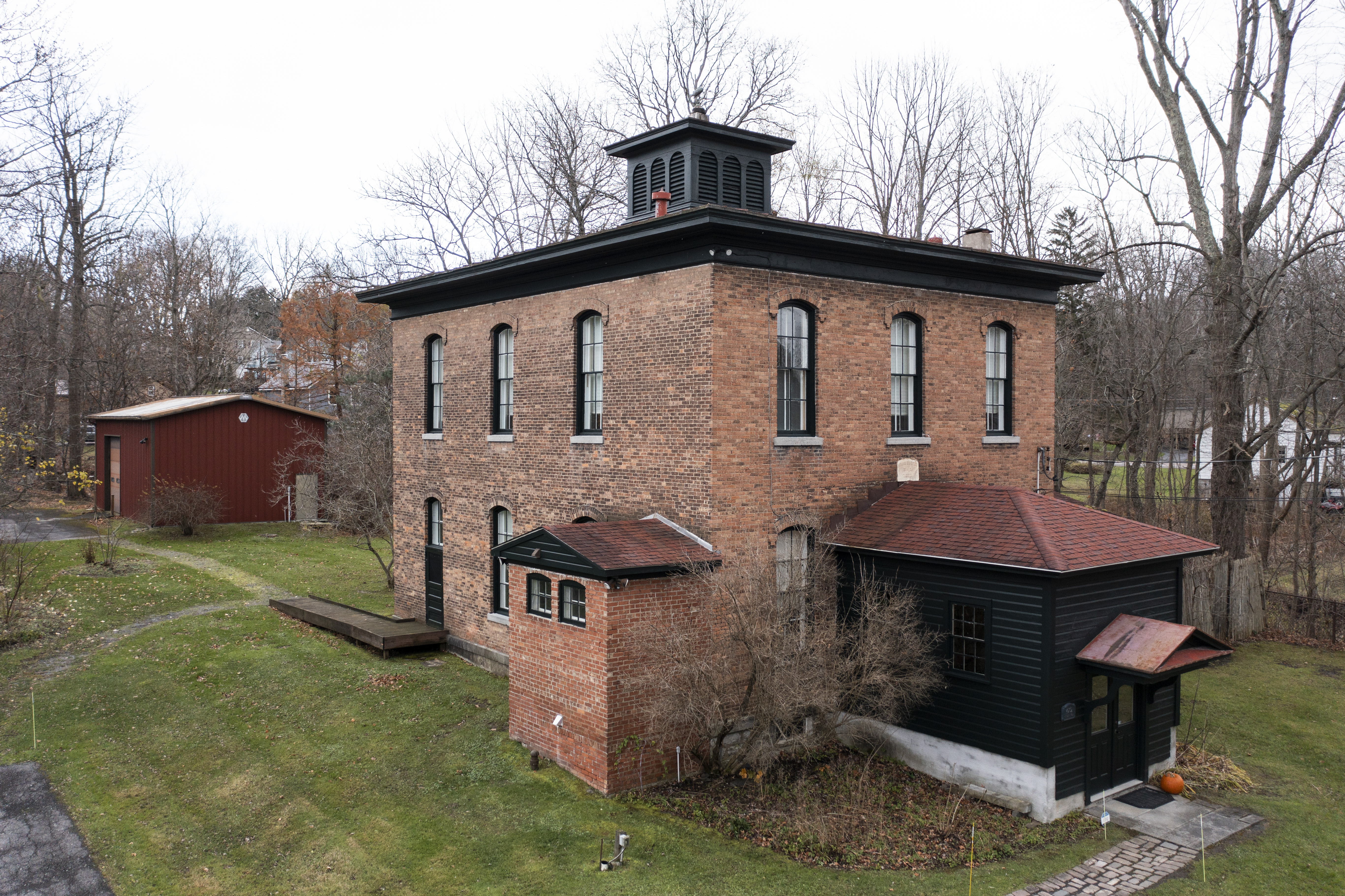This photograph captures a stark, square, two-story brick building set in what appears to be a suburban area, taken during early spring, fall, or winter when the trees are bare. The sky is completely overcast, contributing to the cold and uninviting atmosphere. The grass in the foreground is slightly green, interspersed with pavement on the lower left side and a cobblestone sidewalk that winds around the building, leading to a small porch adorned with an uncarved pumpkin, suggesting it might be close to Halloween. The building features a black roof with a small tower-like structure or possibly a chimney at the top. To the left of the building is a red shed or one-car garage, connected by another pathway. In the background, through the sparse trees, additional houses hint at the suburban setting. The windows of the central building are distinctively curved at the top, and an addition on the back appears to be a black-panel extension that might be a screened-in porch, adding to the uniform yet stark aesthetic of the scene.